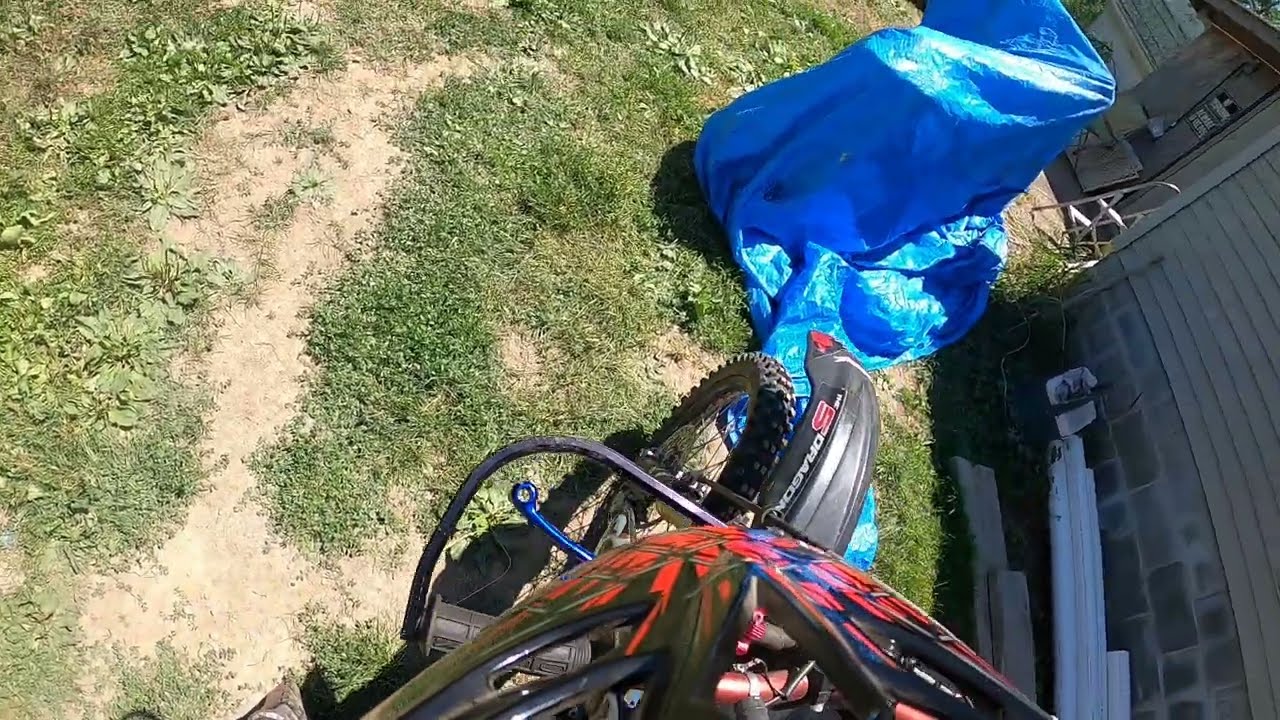In this full-color photograph, taken outdoors on a bright, sunny day, you see a scene captured from the perspective of a rider on a dirt bike, likely with a camera mounted on their helmet. The horizontally rectangular image features the bike's black front fender and tire prominently in the foreground, along with a hint of red accents on the vehicle. The ground below is a messy mix of grass, weeds, and dirt, typical of an untended backyard trail.

To the right side of the image, there's a house with a combination of cinder block and vinyl siding. attached to this building are signs warning "No Trespass" and "Beware of Dog." In front of the motorbike, a blue tarp covers what seems to be another motorcycle based on the shape. Nearby, there is a small white two-step ladder, adding to the cluttered appearance of the scene. The overall perspective and composition hint at this being part of a video likely shot with action camera equipment, capturing the rugged and unrefined surroundings in detail.